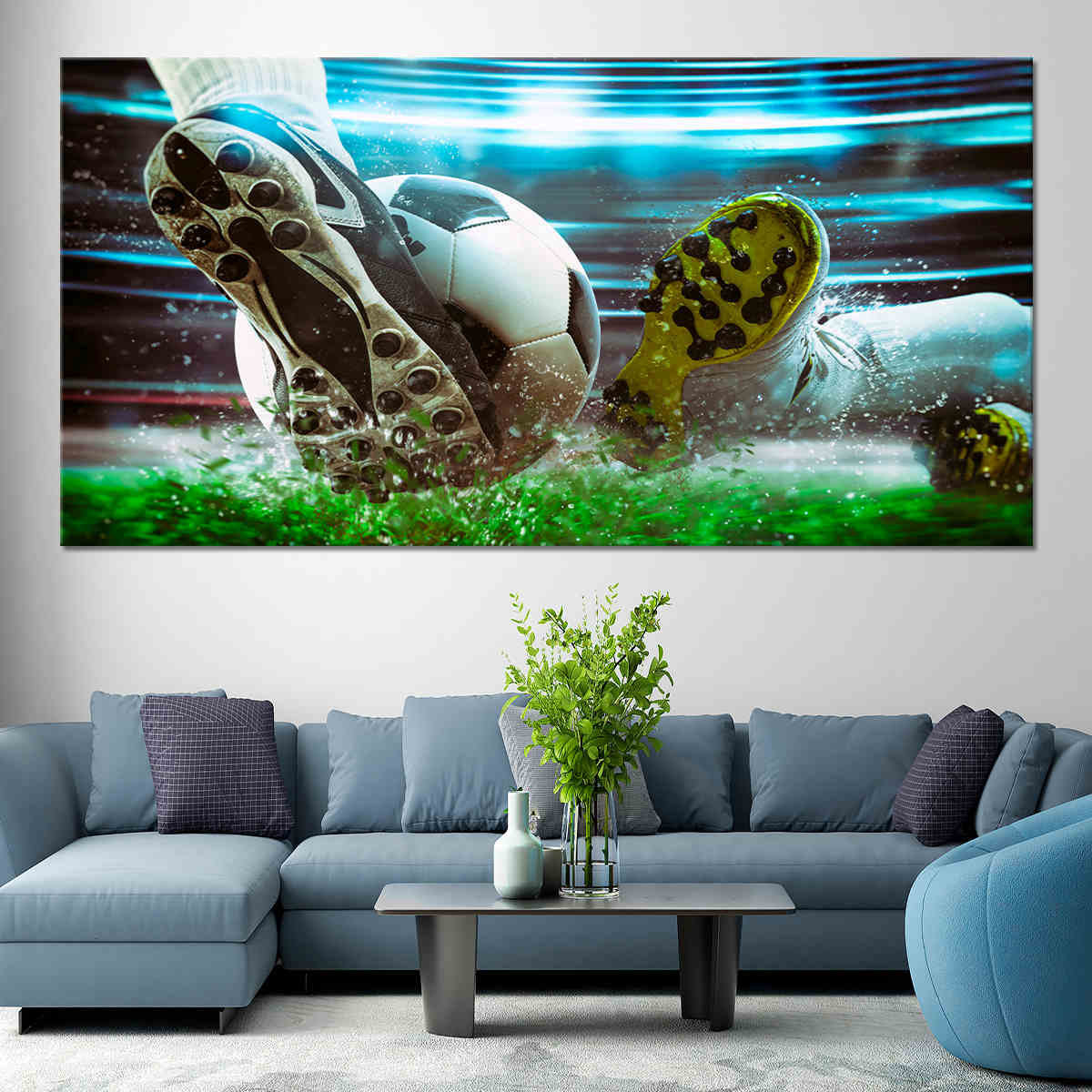The photograph captures a meticulously arranged living room scene, centered around a blue c-sectional couch adorned with a variety of cushions, including matching blue pillows and some in a navy and white checkered pattern. The left side of the couch features an attached chair, seamlessly blending into the sectional design. Positioned in front of the sofa is a sleek coffee table crafted from silver metal, which holds a tall glass vase with lush green leaves and an empty, white ceramic vase beside it. To the right of the coffee table sits a uniquely shaped, donut-like blue accent chair. The entire seating arrangement rests on a light gray area rug featuring a distinctive darker gray pattern. The backdrop consists of a light gray wall, highlighted by a large, rectangular photograph in a landscape orientation. This striking image showcases the dynamic moment of two soccer players' feet—one player's yellow-soled shoes and the other's white shoes with grass-gripping material—jostling for a soccer ball, set against a blurred blue and black background that suggests the intensity of the game. The lower portion of the photograph depicts a patch of grass, grounding the action within a stadium setting.